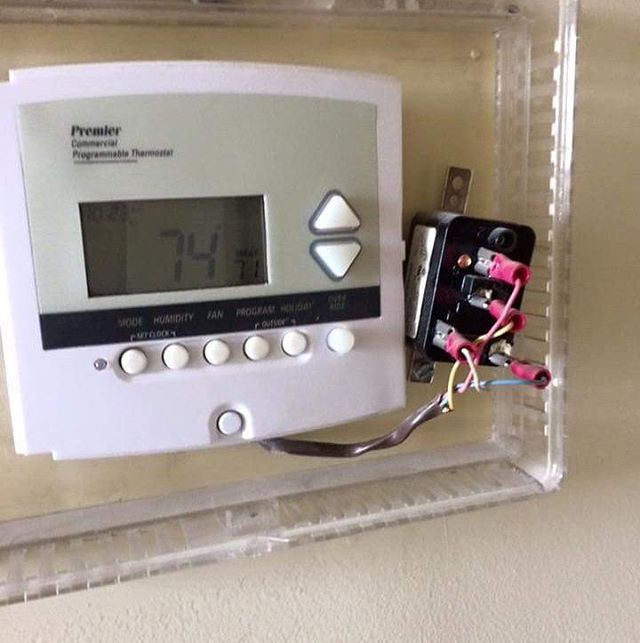A close-up image showcases a digital thermostat mounted on a white wall. The thermostat is powered on, displaying a large, centered temperature reading of 74°F on its main screen. In the top left corner of the display, the time is shown as approximately 10:20 a.m., evident from the well-lit ambiance. The bottom right corner features smaller text and a secondary temperature reading of 71°F. Adjacent to these readings are up and down buttons for adjusting the temperature. Below the main display, there is a row of six additional buttons. A visible cord extends from the bottom of the thermostat, connecting to a series of interrupters or fuses on the right side. The entire device is encased in a transparent plastic frame.